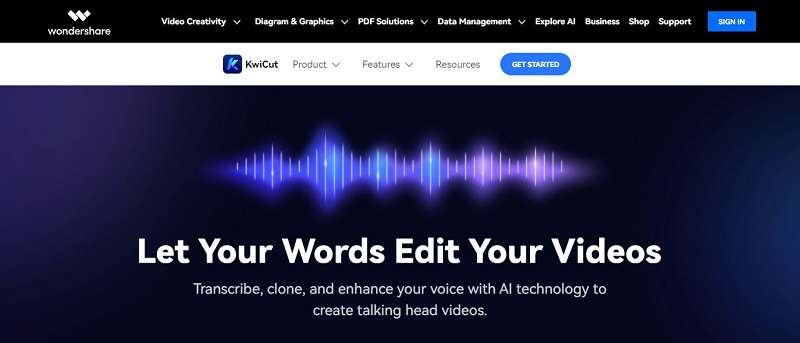The interface for Wondershare features a sleek black horizontal banner at the top. Positioned on the left side of the banner is the Wondershare logo, which consists of three tilted rectangles forming a stylized "W." The word "Wondershare" is displayed in white text below the icon. To the right of the logo, there are four bold-lettered dropdown tabs labeled as "Video Creativity," "Diagram & Graphics," "PDF Solutions," and "Data Management." Further to the right, additional options such as "Explore AI," "Business," "Shop," and "Support" are listed. At the far right end of the banner is a blue, rectangular "Sign In" button with white text.

Separating the banner from the content below is a white space. Beneath this space is a smaller interface element showcasing "Kiwi Cut," which is highlighted by a blue and purple square bearing the letter "K." Beside this, gray text options are labeled "Product" (with a down arrow), "Features" (with a down arrow), and "Resources." Accompanying these options is a blue, oval-shaped "Get Started" button with white lettering.

The main image below these options is a horizontal rectangle that smoothly transitions from purple on the left to gray on the right. Superimposed on this gradient background are dynamic sound waves, displayed in shades ranging from purple to pink, adding a sense of motion and vibrancy to the visual presentation.